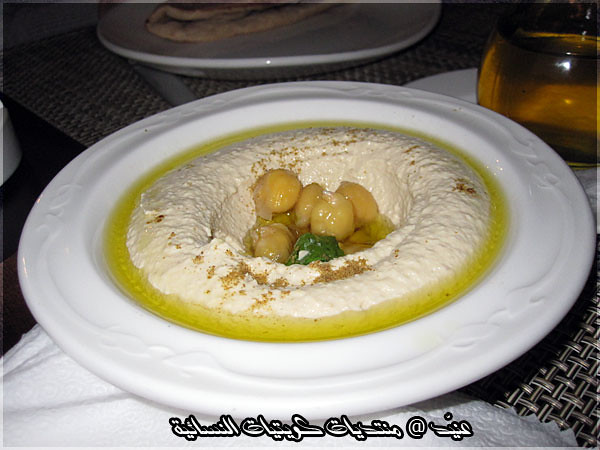This photograph captures a detailed scene featuring a white, round plate, resembling a shallow bowl with a slight hollow in the center, on a black and white woven placemat with a paper towel underneath. The dish appears to be creamy hummus, topped centrally with several garbanzo beans, a hint of brown sprinkles, and a single green mint leaf. The hummus is encircled by a glistening ring of oil, creating a vibrant contrast. The background reveals a glass bottle of oil and another plate with what looks like a folded piece of chicken. The entire presentation rests on a table with gray matting, and there is some text in a foreign language at the bottom of the photograph.